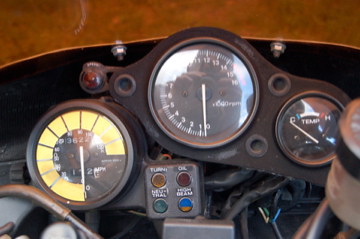The image depicts a dashboard of a classic vintage car, predominantly featuring a dark brown color. The design is uniquely characterized by a metal overlay that slightly arches over the dashboard. The instrumentation panel is adorned with several circular gauges that evoke a nostalgic charm with their retro styling.

On the left side, there's a gauge with a red indicator, likely signaling an issue with the engine. Centrally located is the speedometer, which displays the vehicle's speed in a counterclockwise direction ranging from 0 to 160. Below the speedometer is a temperature gauge marked "Temp" with designations from 'C' (Cold) to 'H' (Hot), highlighted by a gradient from blue near 'C' to red near 'H', signifying temperature levels. The middle of this gauge features a white line to assist in reading the temperature.

On the far right, another round gauge presents, divided into numerous yellow sections and serves to display the vehicle's mileage. The outer perimeter of this gauge is lined with yellow squares, while the middle section provides mileage readings.

Additionally, the dashboard includes a series of small indicator lights in various colors - yellow, red, green, and blue, each corresponding to different vehicle alerts such as oil pressure (red) and other maintenance signals. A tangle of wires is visible beneath the dashboard, hinting at the car's aged, perhaps lovingly maintained, condition.